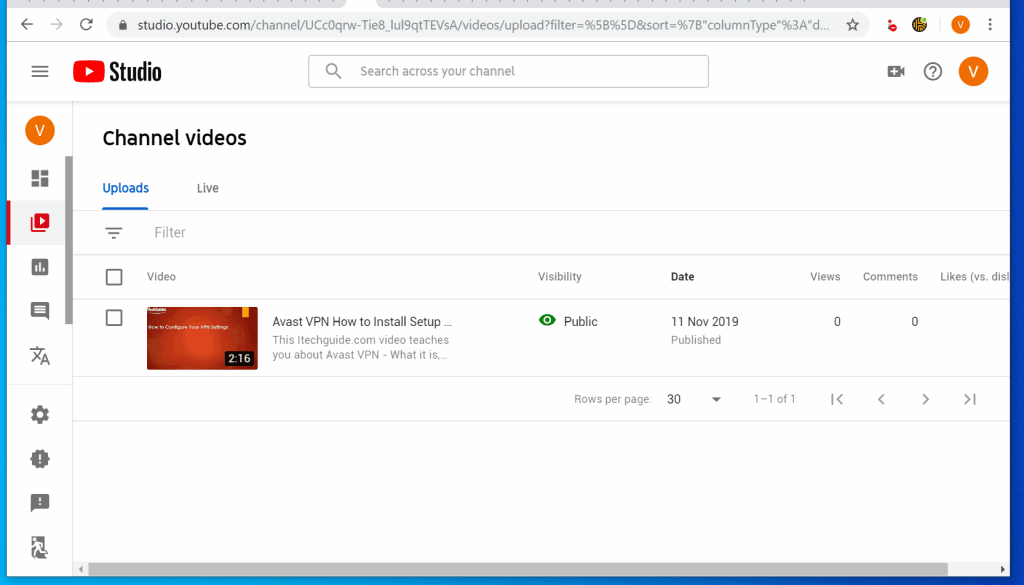A detailed screenshot from YouTube Studio displayed in a Google Chrome browser. At the very top, various Chrome elements are visible: the back, forward, and refresh buttons, alongside a lock icon indicating a secure website. The URL in the address bar reads: `studio.youtube.com/channel/UCcOoQrw-Tiee_lUL9qtTevSAvideo/logout?filter=[filter text]`. There is a bookmark icon next to the address bar.

Below the browser address bar, the YouTube logo and the words "YouTube Studio" are located at the top-left corner with the distinctive red play button. Towards the top-right corner are three icons: a plus symbol to add videos, a question mark for help, and a circular 'V' icon representing the user's avatar.

In the middle of the screen, the title "Channel Videos" is displayed in bold black text. Directly beneath it are two tabs: "Uploads" (highlighted in blue as the current selection) and "Live" (in grey). Below these tabs is a filter dropdown option.

The main content area displays a table with columns labeled as: Video, Visibility, Date, Views, Comments, and Likes. The first row under the columns shows a video thumbnail featuring red coloring and text reading "2:16 Avast VPN How To Install Setup". Accompanying text below the thumbnail reads: "This ITechGuide.com video teaches you about Avast VPN – what it is, what it does..."

Under the "Visibility" column, a green eye icon and the word "Public" are visible. The "Date" column shows "11 Nov 2019", while both "Views" and "Comments" columns indicate "0". Towards the bottom of the page, it indicates that the settings display "Rows per page: 30" with only one video on the current page (1 of 1).